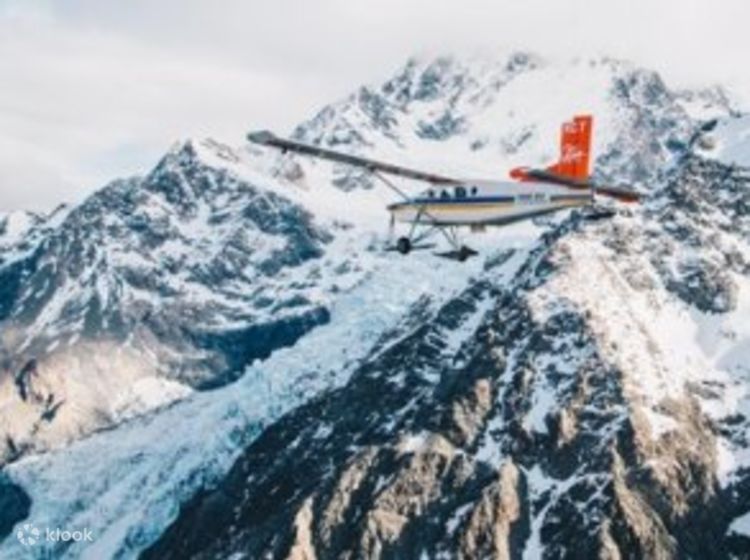The photograph captures a small, private airplane in mid-flight, taken from an aerial perspective. The mostly white aircraft, adorned with a blue and yellow stripe along its fuselage and a red tail, is flying very close to snow-capped, grey mountain peaks. The airplane's landing gear is visible, indicating that it may be preparing to land. The image is somewhat blurry, making the blue letters on the side of the plane hard to decipher, though "Lab" appears to be part of the text. The overcast and foggy sky adds to the dramatic setting. In the bottom left corner of the image, the word "KLOOK" along with a logo is noticeable.